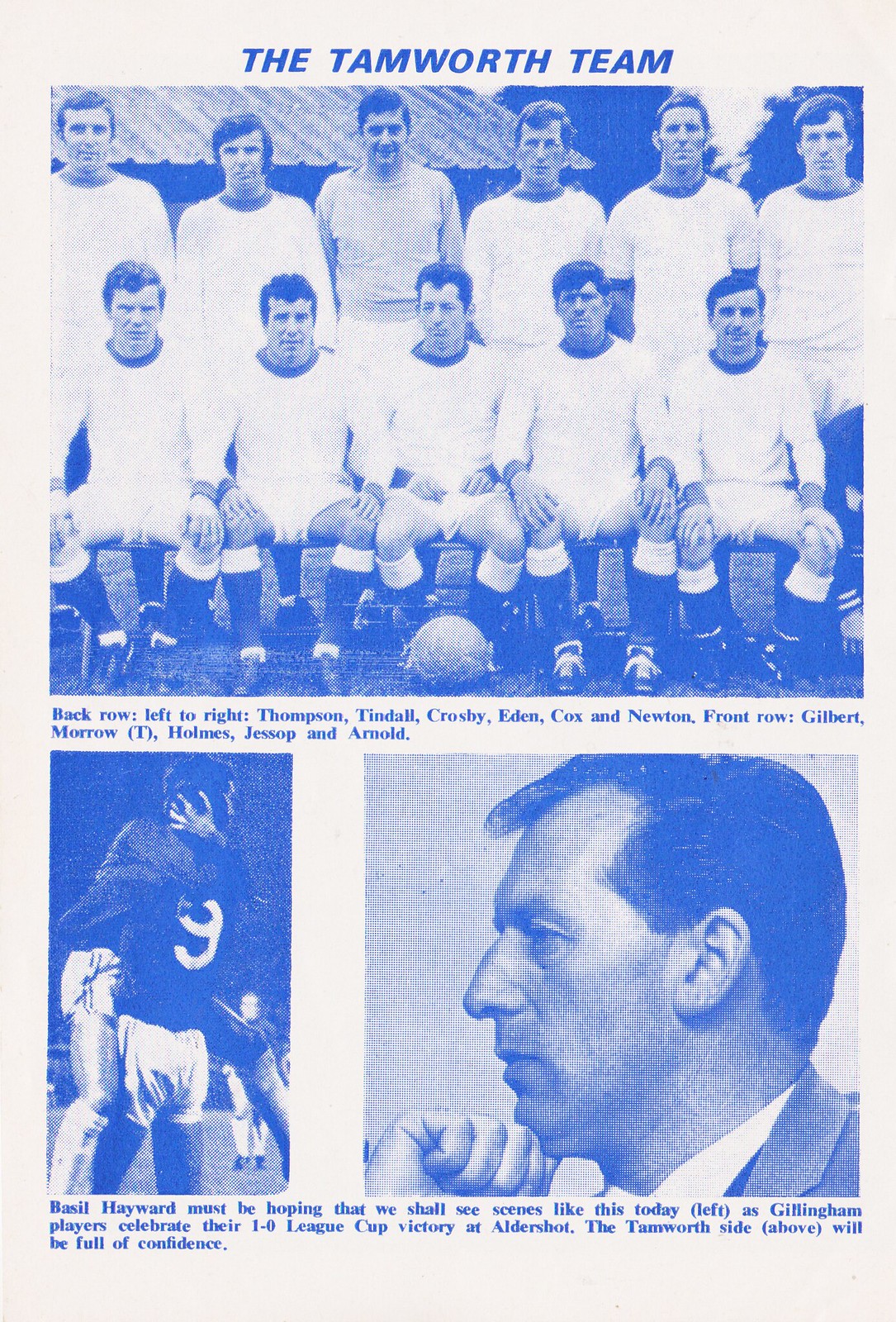This image features a vintage magazine page, primarily in shades of blue and white. Dominating the top is the title "The Tamworth Team." Below the title is a classic black-and-white photograph of a soccer team, although the blue hue can make it hard to distinguish exact colors. The image portrays two rows of men; the back row is standing, and the front row is seated, all in what appears to be white jerseys and shorts with a soccer ball placed in front of them. Identifications for the players are provided beneath the photograph: back row from left to right includes Thompson, Jindal, Crosby, Eden, Cox, and Newton; front row from left to right lists Gilbert, Morrow, Tee, Holmes, Jessup, and Arnold.

Beneath this team photo are two additional images. The first shows two players embracing, one of whom has the number nine on his jersey. The second image depicts a man in a gray suit staring to the left with his hand resting under his chin. Accompanying these images is a caption in blue text on a white background: "Basil Hayward must be hoping that we shall see scenes like this today as Gillingham players celebrate their 1-0 League Cup victory at Aldershot. The Tamworth side will be full of confidence." The overall composition and details suggest this is likely a page from a sports yearbook or magazine.